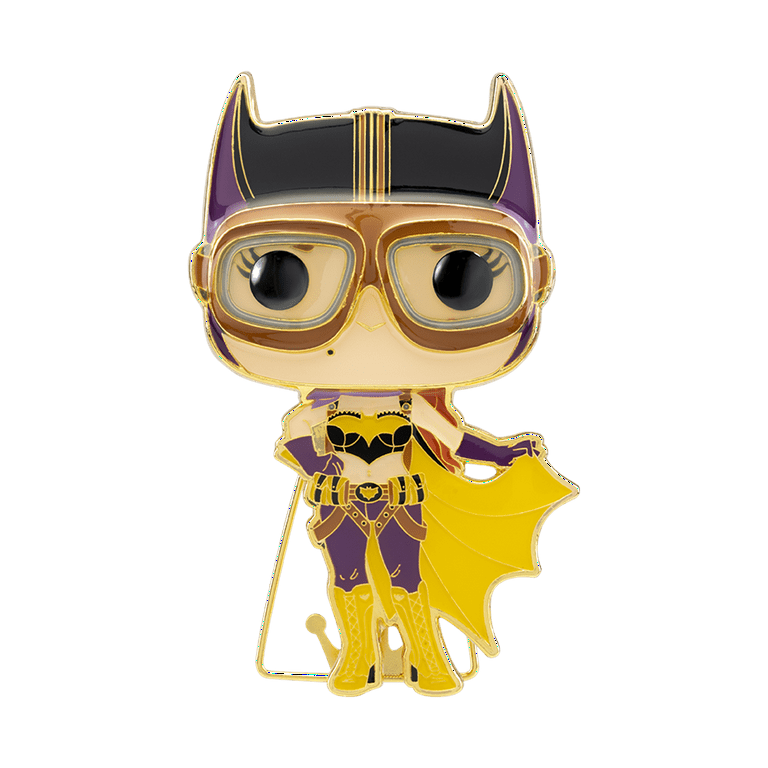The image features a cartoon character resembling a cross between a Pop Funko figure and a superhero caricature. The character has an oversized head, almost bobblehead-like, with large black eyes and no mouth. Sporting a black and purple helmet with ear-like horns and yellow striping, the character also wears thick brown goggles that resemble aviator glasses. 

Her outfit consists of a gold and black bralette, purple pants, and yellow boots. She accessorizes with purple gloves and a gold and black belt. A gold cape flows to her right, held out dramatically by her outstretched arm. The character's design is outlined in a shiny gold color, adding to the superhero aesthetic, and she stands against a white background. The overall look draws inspiration from iconic superhero designs, possibly reminiscent of Batgirl or Cat Woman.